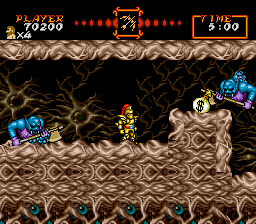This screenshot is from a retro-style, pixel art video game, characterized by its 2D graphical appearance. At the center, the main character, adorned in a gold suit of armor with a distinctive red plume or hair emerging from their helmet, stands poised. To the character's right, a small mound obstructs their path. Atop this mound, a bag emblazoned with a dollar sign promises potential treasure.

Flanking the protagonist on both sides are two nefarious enemies. These adversaries possess blue skin and are outfitted in purple garments – possibly overalls and mittens. Each wields an axe, either brass or gold in color, menacingly aimed at the main character.

The backdrop of the scene is stark black, enhancing the vibrant colors of the characters and objects. At the top of the screen, "Player" is prominently displayed in red, with various stats beneath it detailing the protagonist's status. In the center, an icon indicates the character's current weapon, which appears to be a metallic bow. On the far right of the screen, a timer, displayed in white, reads five minutes, adding a sense of urgency to the scenario.